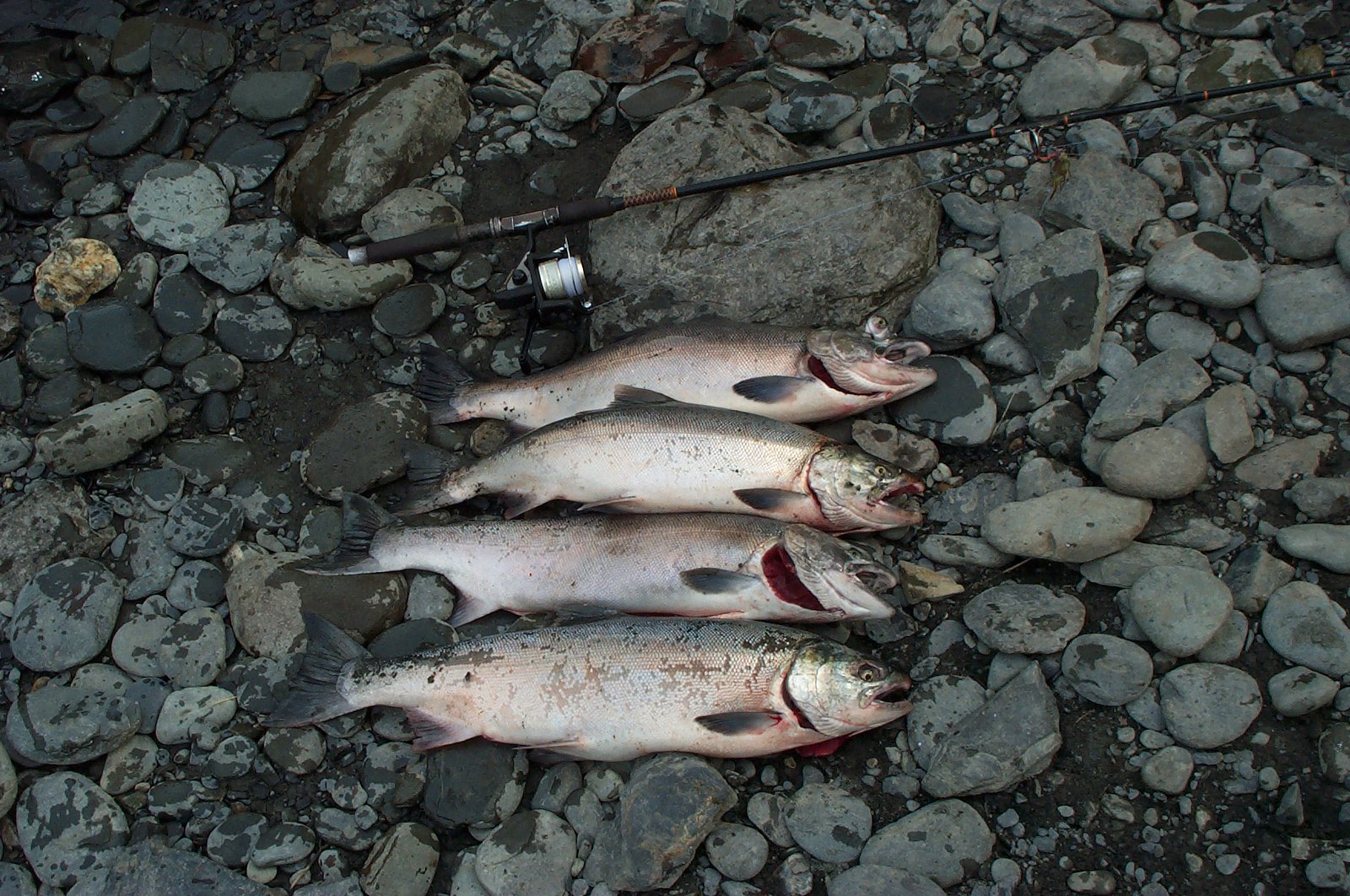This outdoor photograph showcases four caught fish lying in a neat row on a bed of dark gray, rounded stones with noticeable discolorations from water splashes, suggesting their recent retrieval. Each fish, displaying a shiny silver skin and characterized by open mouths facing right and dark-colored tail fins to the left, shares a distinctive small gray fin behind the gill slits, hinting at a salmon species. Positioned above the fish is a black fishing rod extending diagonally to the upper right of the image. The rod, resting on a larger central rock, features horizontal orange lines and a silver and white reel situated closer to the fish. The scene is detailed with a mix of variously sized rocks, including a notable yellowish-golden one at the far left, adding depth to the natural setting.